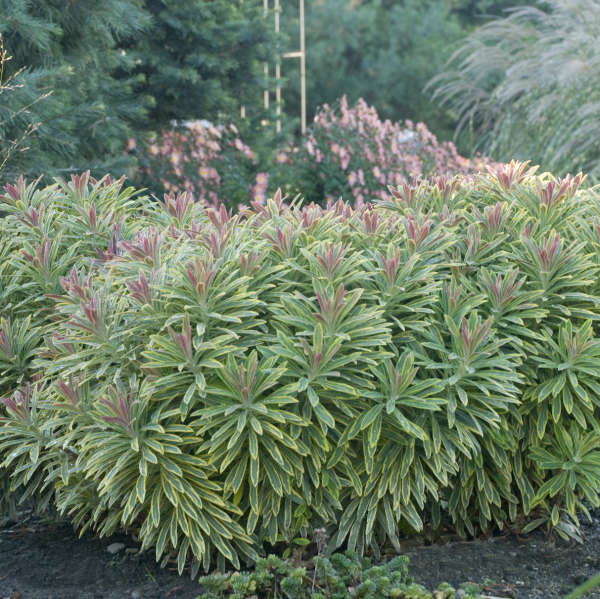This outdoor photograph captures a lush garden scene dominated by vibrant greenery and burst of colors. At the centerpiece is a strikingly large, green bush characterized by variegated green and yellow leaves, with pinkish-red tips that resemble new growth. Surrounding this main plant are additional green bushes, some displaying similar red and pink-tipped leaves and others adorned with pinkish flowers or budding blooms. The ground beneath these plants is covered with brown mulch that keeps the area moist and is interspersed with dark, rocky volcanic-like soil. In the background, which is blurry, one can discern taller trees that may be pine or some other kind of tree, and a wooden structure with thin pieces visible, possibly a trellis. The scene paints a vivid picture of an intricate garden with diverse plant life captivating the viewer’s attention.